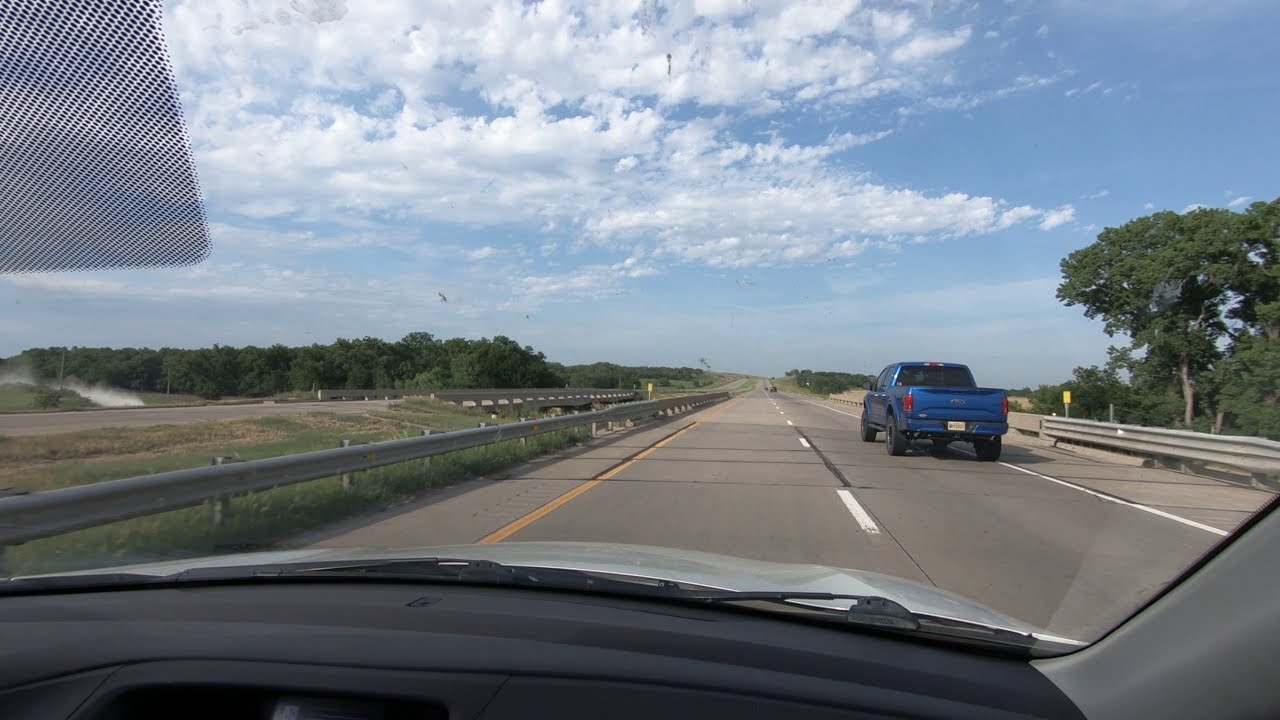The photograph, taken from the passenger seat inside a car driving north on a highway, captures a detailed view of the road and its surroundings. The vehicle is on a multi-lane, light gray asphalt highway, delineated by a dotted white line marking lanes, with solid white lines on the outer edges and a yellow line on the interior side. Ahead is a blue pickup truck with tinted black windows traveling in the same direction. To the left, a separate, distant lane for opposite traffic is visible, divided by ramps, a spacious grassy field, and green trees that line both sides of the road. Wooden posts with a gray metal railing provide additional safety barriers. The scene unfolds under a daytime sky characterized by a mix of light blue and numerous white clouds, with some white smoke visible in the far distance to the left.